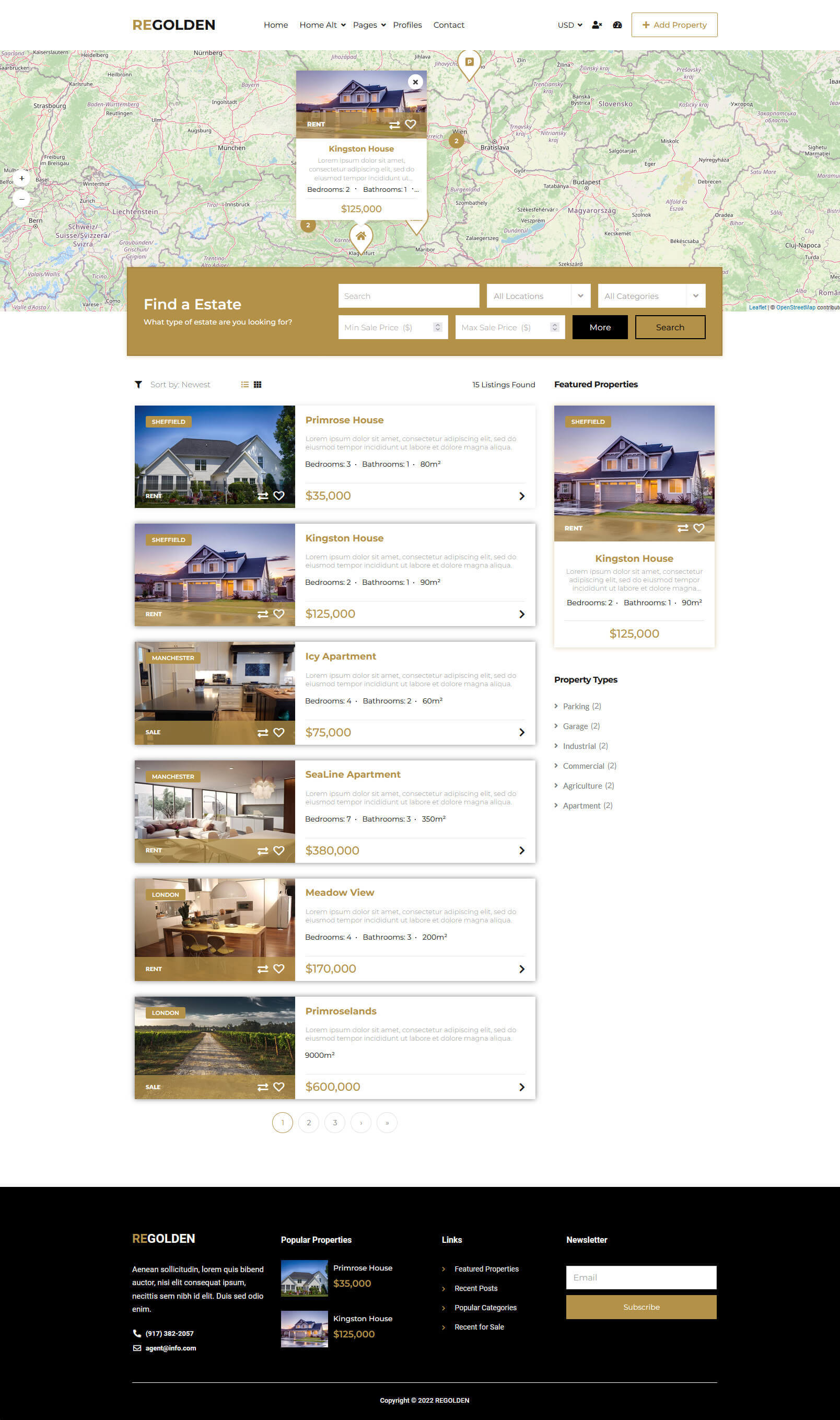Screenshot of ReGolden Real Estate Website Mock-Up:

This detailed screenshot captures the entirety of a real estate website from top to bottom, showcasing a mock-up likely created from a template. At the very top is the logo "ReGolden", with "R" highlighted in gold and the rest in black. The navigation menu includes links such as "Home," "Pages," "Profiles," "Contact," along with currency options (US dollars) and a section to add a property.

At the top section, an embedded Google map displays several property markers, with the mouse hovering over one labeled "Kingston House," accompanied by a photo of a house at sunset. This listing includes details mentioning it's a three-bedroom, one-bathroom property priced at approximately $125,000, with an option to rent.

Below the map, there is a search functionality labeled "Find Estate," featuring fields to search by categories, locations, price range, and additional parameters. This area allows users to refine their property search based on their preferences.

The main content area presents six property listings. The first property, "Primrose House," is priced at $35,000, offering three bedrooms and one bathroom with an approximate size of 80 square meters. Following that, "Kingston House," details three bedrooms and one bathroom, spanning 90 square meters, and priced at $125,000.

The subsequent listings showcase internal shots of various properties such as "IC Apartment" and "C-Line Apartment," followed by "Meadowview" and another "Primrose" listing. The final listing depicts an agricultural scene with a road bisecting the crops.

Adjacent to the main listings, a "Featured Properties" section reiterates details of highlighted properties like "Kingston House." Property types are categorized on the side menu, including options such as parking, garage, industrial, commercial, agricultural, and apartments.

At the bottom of the page, navigation options include pagination controls for browsing additional property pages. The black footer contains links to popular properties, additional navigation, and a sign-up area for the newsletter.